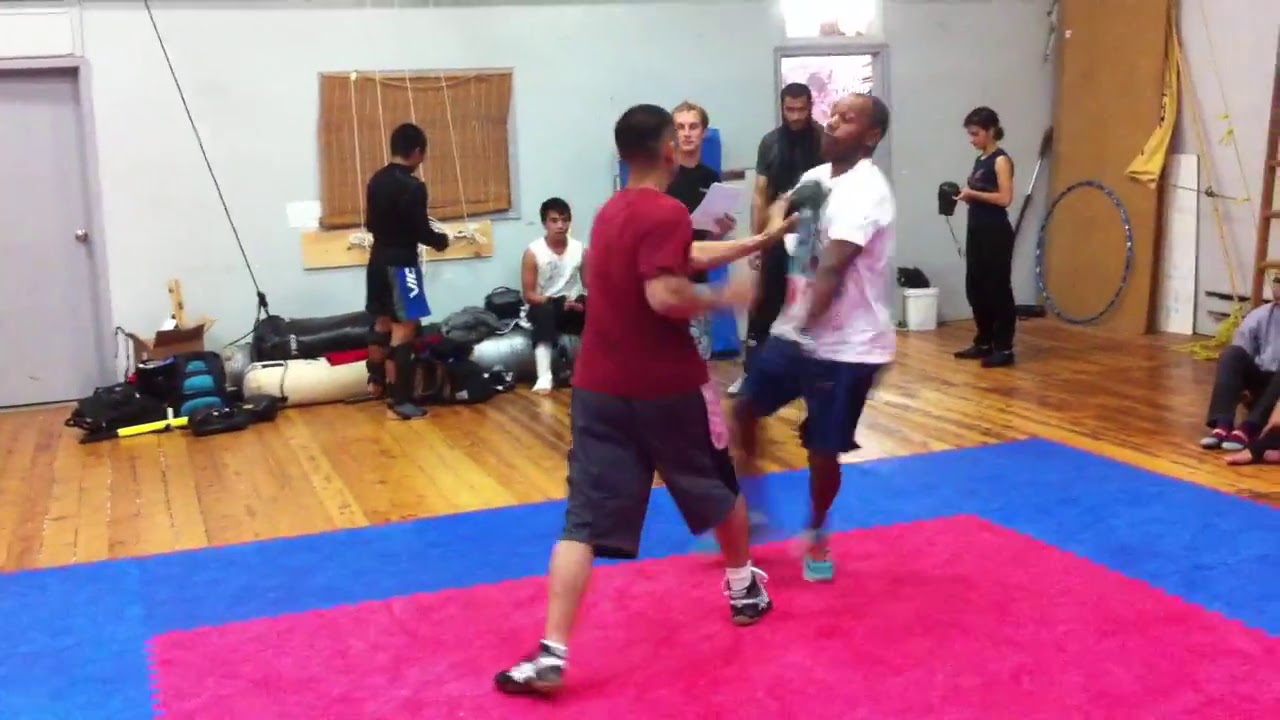In the photo, a lively scene unfolds inside a building with hardwood floors. Two men are engaged in a physical altercation on a large mat that spans from the lower left to the middle right, and down again to the lower right, featuring a vibrant blue and hot pink design. The man closest to the camera wears a red t-shirt and black shorts, forcefully pushing the other man, who is dressed in a white t-shirt and blue shorts, causing him to tumble sideways. Surrounding them, approximately half a dozen people are either observing the scuffle or engaged in their own activities. The background features a white wall adorned with various colored gym equipment, including white and black mats, and blue gear. A white door and a small white trash can are also visible, adding to the indoor gym setting. One of the windows has its blind down, while another window is partially obscured by an onlooker.